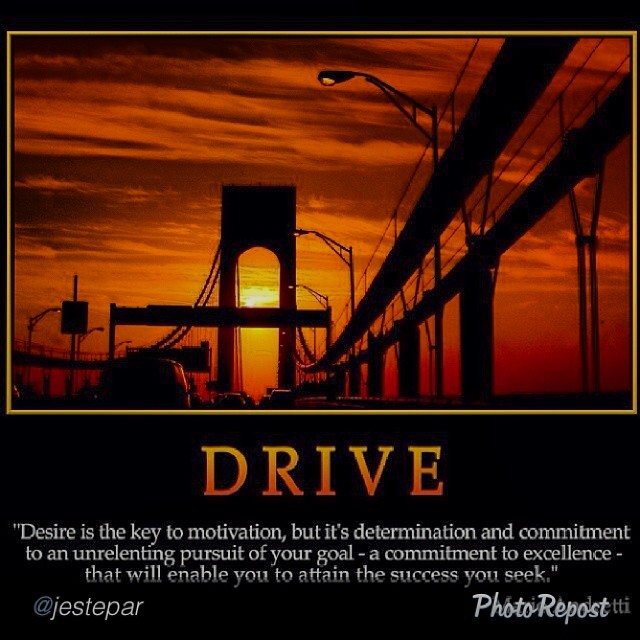The image is a poster with a black background and an evocative depiction of a bridge at dusk. The upper portion of the poster, which occupies about 60% of the space, features a digital image of a long bridge. The scene includes a dark, orange sky with clouds tinted by the setting sun, and shadows cast over the bridge, which appears black. In the center of the image, the sun sets under an arch of the bridge, creating a striking contrast. Dark silhouettes of cars are visible on the bridge, as well as indistinct road signs and streetlights lining both sides.

Beneath this image, large capital letters in an orange gradient spell "DRIVE." Below this title, in smaller white letters, lies the motivational quote: "Desire is the key to motivation, but it's determination and commitment to an unrelenting pursuit of your goal, a commitment to excellence that will enable you to attain the success you seek." At the very bottom, there are the text identifiers "@J Step R" and "Photo Repost."